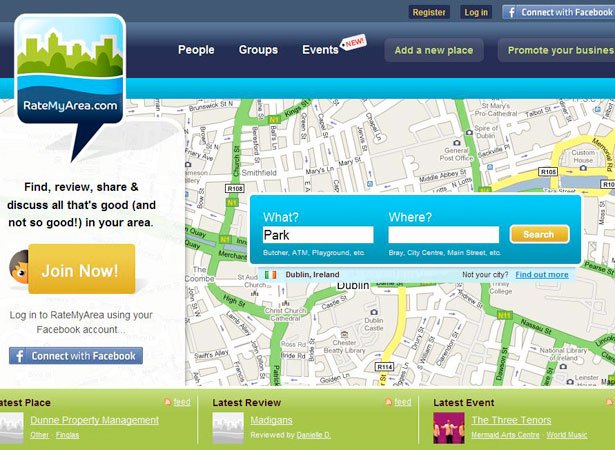Screenshot of RateMyArea.com Website:

This image captures a web page from RateMyArea.com, an online platform designed for locating and rating various places around the world. The central focus of the page is a large blue box that sits prominently in the middle, offering fields labeled "What" and "Where" for conducting searches. In this instance, the search query is for a park in Dublin, Ireland. 

In the background, the page features a map displaying the Dublin area, providing geographical context for the search. Just below the search box are three green-highlighted sections showcasing the latest places, reviews, and events in Dublin, giving users up-to-date information about the area. This helps users find not only parks but also other points of interest and community activities.

On the left sidebar, there are options for users to join the RateMyArea.com community and to connect with the platform via Facebook, encouraging social interaction and membership growth. 

Overall, the design of the website appears noticeably outdated, reminiscent of early 2000s web aesthetics, yet it aims to be a valuable resource for both locals and visitors seeking to explore and evaluate different locations.